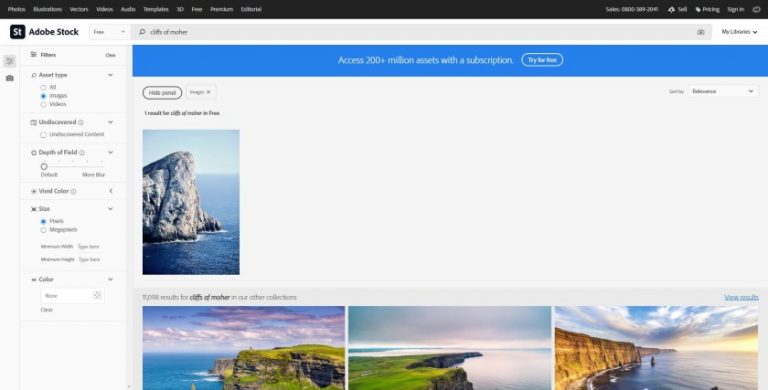A semi-blurry screenshot is captured in this image, which features a dark black header running across the top of the screen adorned with a series of menu items rendered in white text. Although the text is indistinct, it spans the entire header from the left to the right. Directly beneath the header lies a white banner showcasing the words "Adobe Stock" in dark print, accompanied by a small logo featuring a black box with a white "ST" inside it, positioned on the left side. Adjacent to the logo, on the right side of the banner, is a search box. Below this, a vibrant blue banner with white text stands out, reading: "Access 200+ million assets with a subscription." To the right of this statement, there is an inviting blue action button labeled "Try for free." Continuing downward, the image displays a collection of four stunning, full-color photographs depicting various scenic daytime views of water, cliffs, and boulders. There are three images aligned horizontally at the bottom and one larger image on the left side, all highlighting the natural beauty captured in each photo.